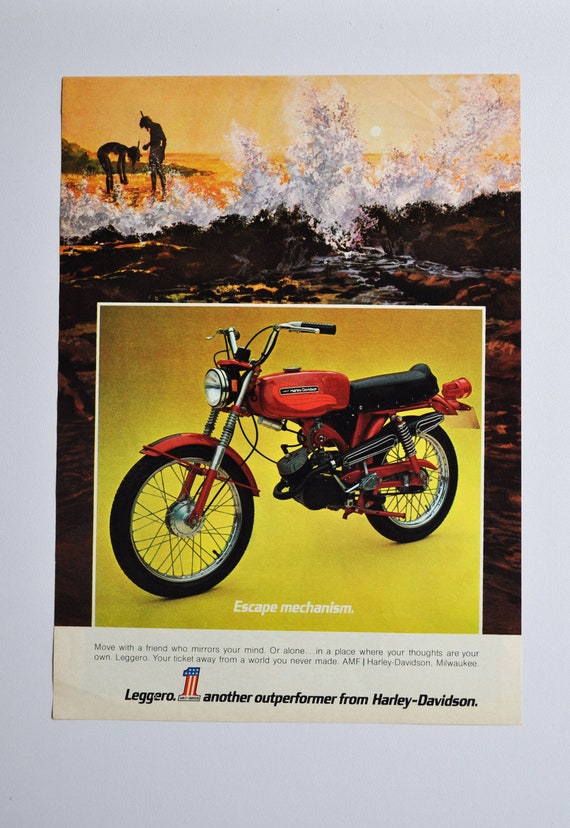This vibrant vintage magazine ad, likely from the late 70s or early 80s, showcases a striking red and black 125cc Harley-Davidson motorcycle, known as the Legaro No. 1. The promotional poster highlights the motorcycle's key features: a red gas tank, front fender, and body, complemented by chrome handlebars and front forks, a black engine and exhaust pipe, and silver rims. The ad's tagline, "ESCAPE MECHANISM," is prominently displayed at the bottom, followed by an inspiring message: "Move with a friend who mirrors your mind or alone in a place where your thoughts are your own. LEGORO, your ticket away from a world you never made. AMF Harley-Davidson, Milwaukee." Set against the backdrop of a scenic beach with waves crashing against the shore and a sun setting in the distance, the illustration also features two young people in snorkel gear, standing in shallow water, adding a sense of adventure and freedom to the alluring imagery.